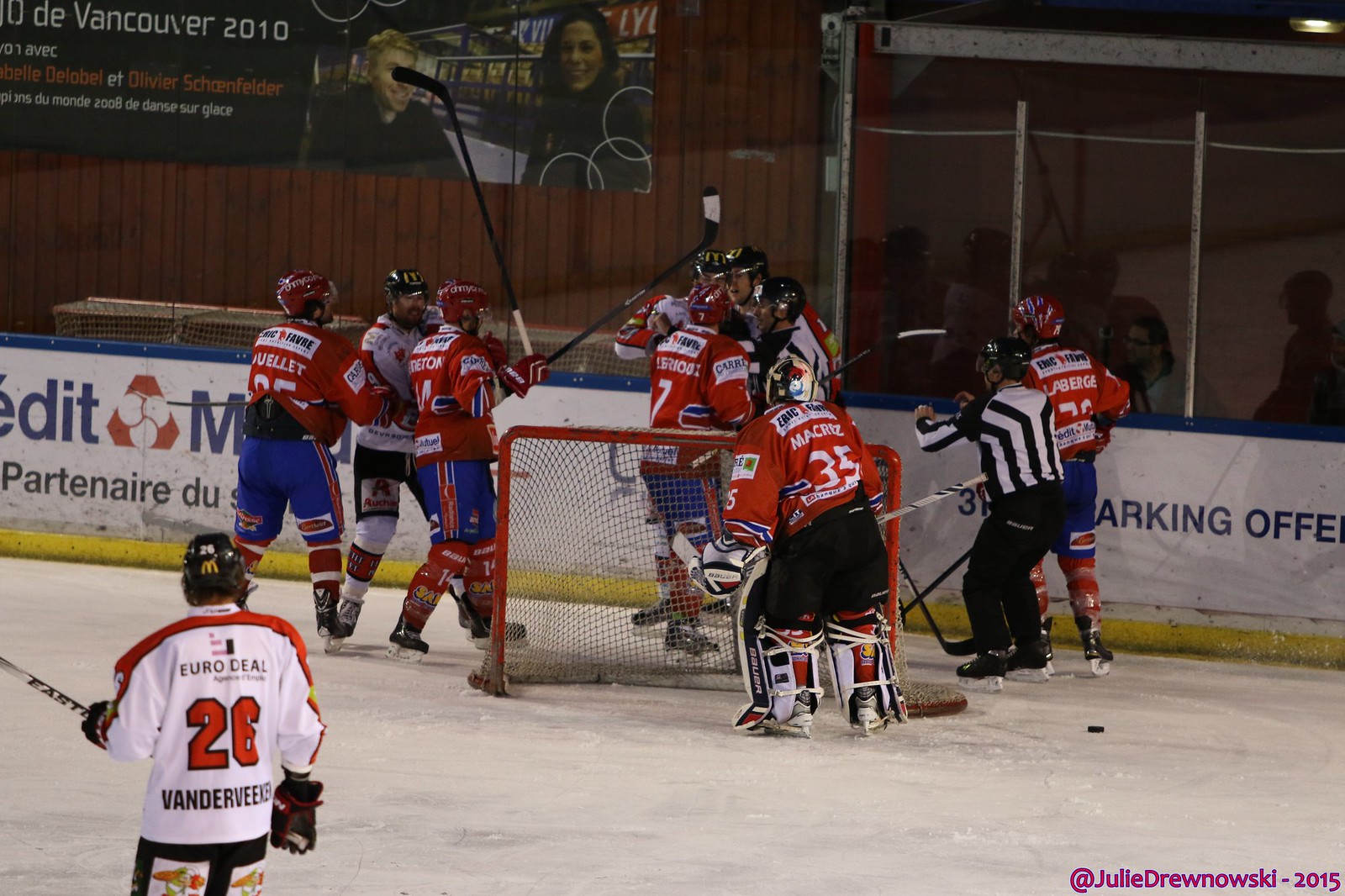This wide rectangular photograph depicts a tense moment during a hockey game, focusing on the goalie area of an ice rink. The bottom half of the image showcases the slightly curved, diagonal ice, bordered by a white barrier. The goal itself is a small, wide rectangle framed with red metal. Behind the goal, several hockey players appear to be in an altercation. Players in red jerseys with blue shorts dominate the scene, while players in white jerseys with orange colors are involved as well. It looks like a skirmish or a celebration of some kind, possibly involving a player from the white team. The goalie in red stands in front of the net, while an official skates into the group, seemingly to break up the commotion. In the lower left corner, a player in a white jersey is noticeable. The wooden plank wall behind the barrier and the large poster in the top left corner set the backdrop for what seems like a minor league game. A "Vancouver 2020" sign indicates the possible location and year. The photo is credited to Julie Grinbrowski, copyrighted in 2015.